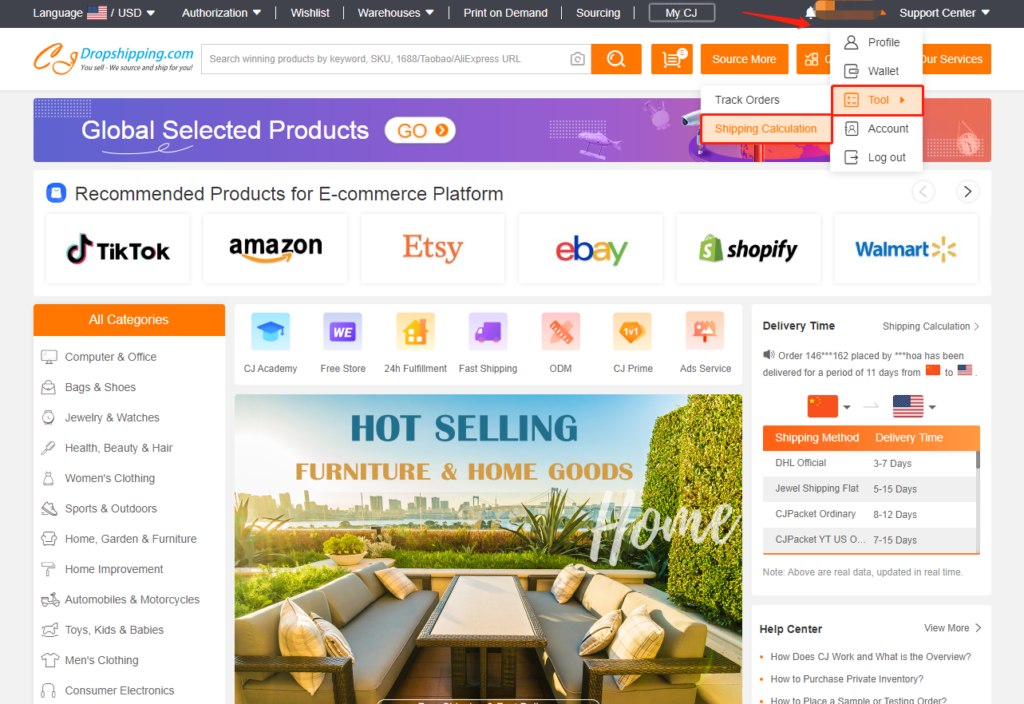The screenshot displays the homepage of CJdropshipping.com, set against a clean, white background. At the top, the site's logo is prominently featured, with "CJ" in orange and "dropshipping.com" in blue. Adjacent to the logo, options for selecting the site language, viewing prices in USD, and accessing sections like authorization, wishlist, warehouses, and print on demand are neatly lined up. Users can also navigate to a personalized area through the "myCJ" link, or get assistance via the "support center."

A striking red arrow points to a dropdown menu under the profile section, highlighting the "wallet two" option, which is enclosed within a red rectangle. The dropdown menu includes additional options such as profile, wallet, account details, and logout. Directly beneath this, a smaller white rectangle contains two further options: "Track Orders" and "Shipping Calculation," with the latter outlined in orange.

At the top of the page, a search bar equipped with a magnifying glass icon invites users to find specific items. Beside it, a shopping cart icon embedded in a white circle displays the number six, indicating the number of items in the cart. Navigation tabs labeled "Source More" and "Our Services" offer further browsing options. 

Prominent category links, including "Global Selected Products," "Recommended Products for E-commerce Platform," and major product categories such as "All Categories," "Computer and Office," "Bags and Shoes," "Jewelry and Watches," as well as "Health, Beauty, and Hair," are visible, each inviting users to explore a diverse range of products tailored for e-commerce solutions.